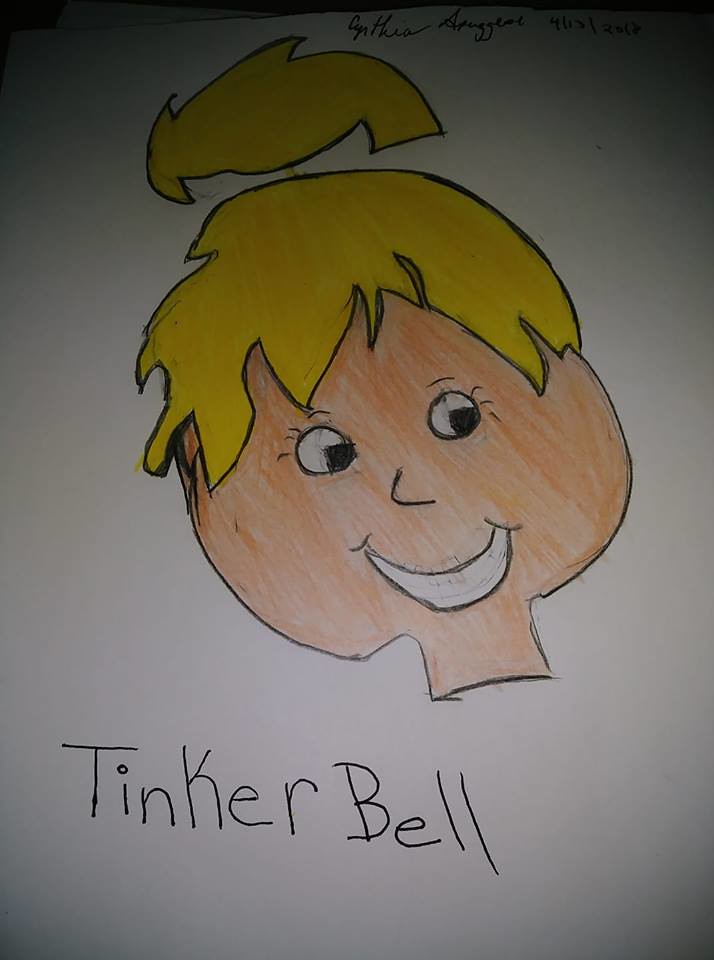The image is a childlike illustration of Tinkerbell's face, drawn on plain white paper. Tinkerbell's head is slightly tilted, resembling a beet with a stem, with shaggy blonde hair gathered in a ponytail or bun on top and some hair falling beside her eyes. Her face is shaded in orange or tan using colored pencil, crayon, or marker. She has round eyes with black pupils positioned towards the bottom right, adorned with three small eyelashes on each eyelid. Tinkerbell's pointy nose is shaped like a sideways V, and she has a white, banana-shaped smile. At the bottom left corner of the image, the name "Tinkerbell" is handwritten in black ink with a capital T and B. Above her head, there is a cursive signature reading "Cynthia Swaggart" alongside the date "4-13-2018." The background of the drawing remains completely white.